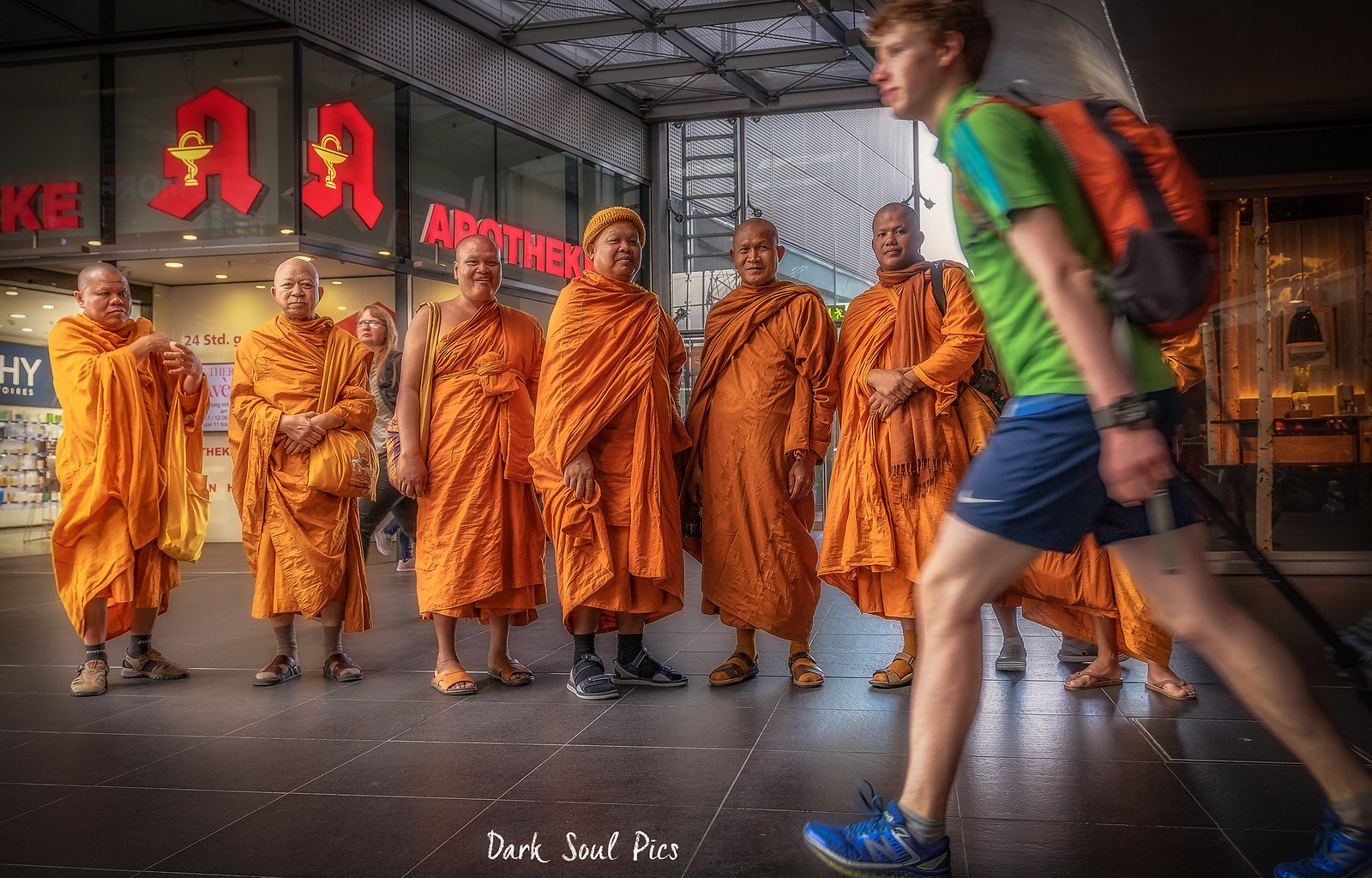The photograph captures a dynamic scene featuring a group of monks and a passerby in an outdoor mall setting. Dominating the image are eight monks of Asian descent, each wearing light orange robes and sandals. All but one have shaved heads, with the exception sporting an orange cap. These monks are standing on a dark brown tiled floor with distinctive white grout lines. In the foreground, a young Caucasian man with short, reddish curly hair is in motion, walking from right to left. He is dressed in a green short-sleeved t-shirt, navy blue Nike shorts, and blue New Balance shoes, carrying an orange and black backpack. He appears slightly blurred, indicating movement, and a pole extends from his hand, suggesting he is pulling luggage. Behind the monks and the man, the background reveals a storefront with a prominent red letter 'A' and the word "APOTHECARY" partially visible. Additional details include items displayed in the store windows and another woman walking in the background. At the bottom of the photograph, the caption "Dark Soul Pix" is elegantly inscribed in small white cursive.